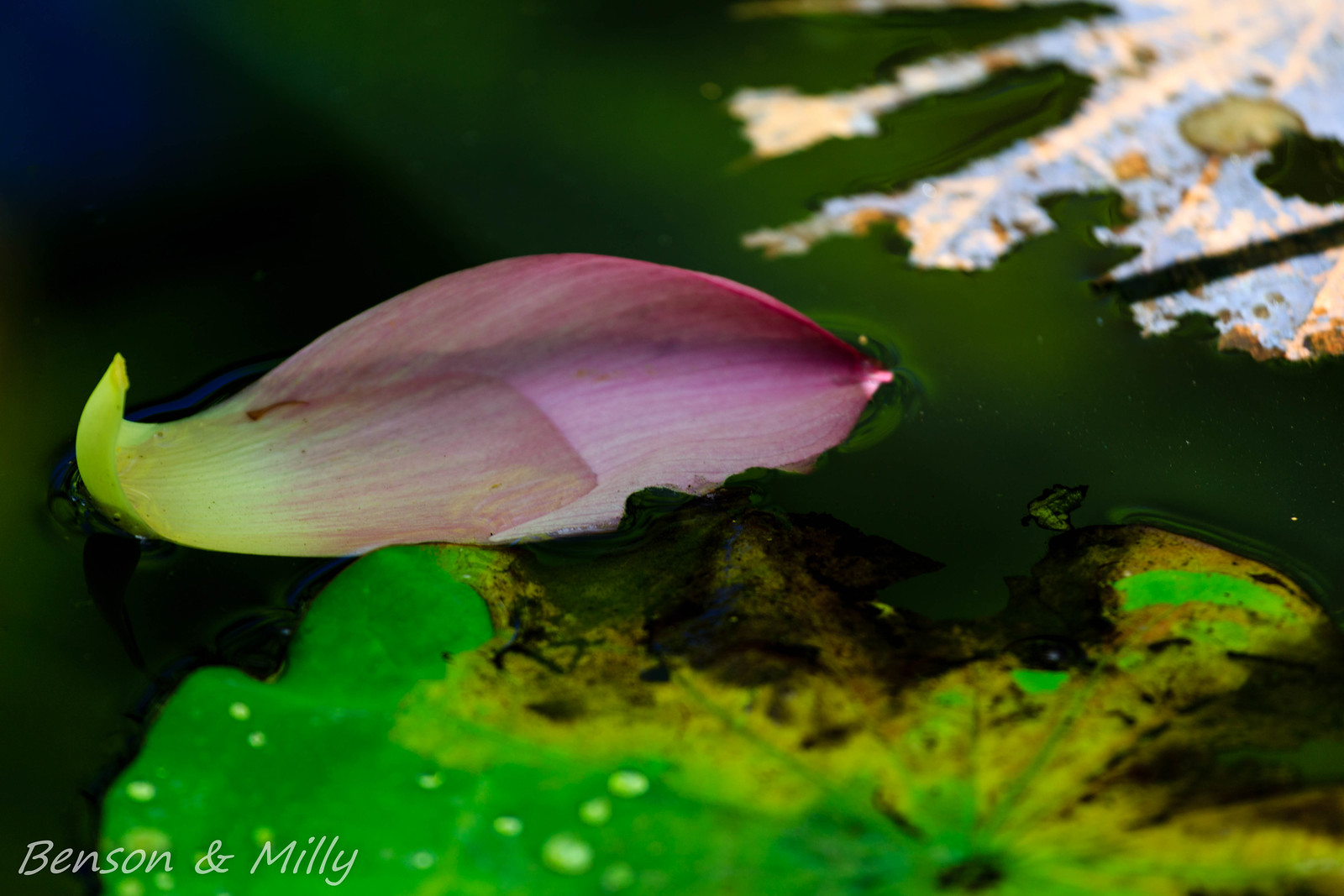This detailed, close-up photograph captures the serene beauty of a lily pond. Dominating the bottom center of the image is a large, vibrant light green lily pad, marked with worn black spots. Directly above it, floating gracefully on the surface of dark green, reflective water, is an exquisite flower petal. The petal displays a striking gradient of colors, transitioning from deep magenta and pink to light green at the tips, which are slightly curled. Positioned horizontally, it serves as the central focus of the photograph. In the top right corner, partially illuminated by sunlight, is a smaller part of another flower, distinguished by its delicate white and gold hues. The entire image is bathed in a green overtint, further enriched by the presence of bright green moss scattered across the scene. Adding a personal touch, the names "Benson and Millie" are inscribed in white letters in the bottom left corner. This captivating image seems to capture a moment of natural tranquility, as if zooming into a peaceful pond filled with vibrant flora.